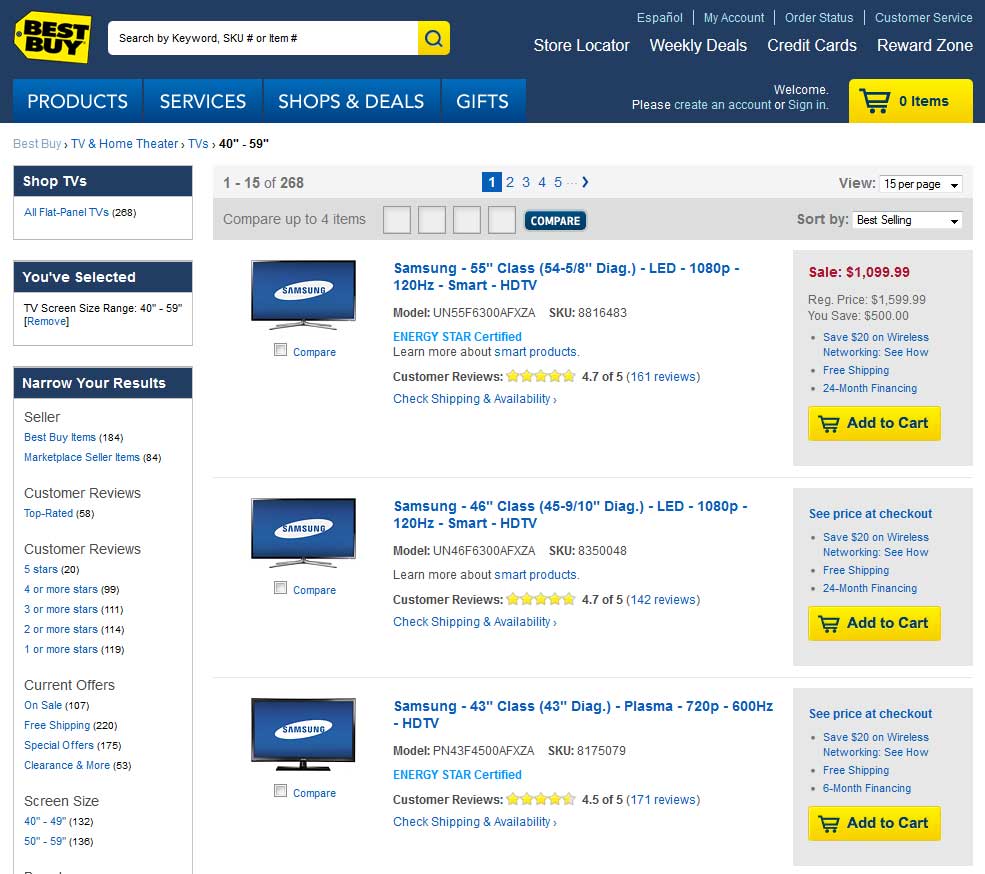In this image, we see a detailed screenshot of the Best Buy website. In the upper left corner, the iconic yellow "Best Buy" logo with dark blue text is prominently displayed. To the right of the logo, the search bar is inviting users to "Search by keyword, SKU, or item number." Just below the search bar, a navigation menu spans horizontally, displaying options labeled "Products," "Services," "Shop Deals," and "Gifts" from left to right. Additionally, there is a yellow shopping cart icon, indicating there are currently zero items in the cart.

The first product listed is a Samsung 55-inch Class LED Smart HD TV (model UN55F6300AFXZA). The precise dimensions are specified as "54 5/8" diagonal. The SKU number for this model is 8816483. To the right of the product description, the sale price is boldly displayed in red: $1,099.99. Beneath the price, a yellow "Add to Cart" button is clearly visible.

The subsequent item shown is a Samsung 46-inch Class LED 1080p 120Hz Smart HD TV. Customer reviews for this model indicate an average rating of 4.7 out of 5 stars, based on 142 reviews. To the right of this product description, instead of a specific price, the text reads "See price at checkout," and it's noted that buyers can save $20 on wireless networking with this product.